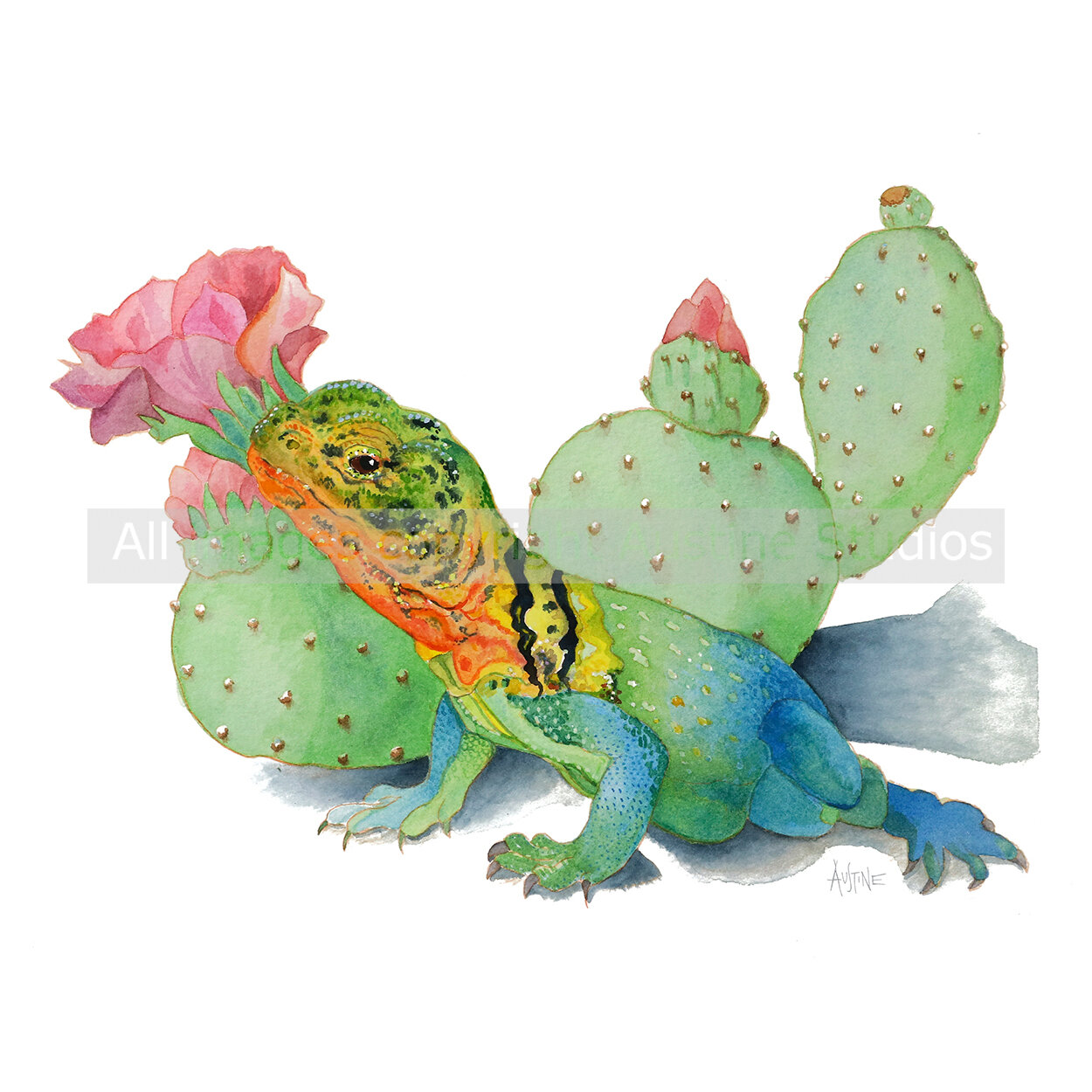The image is a detailed painting, possibly using watercolor or colored pencils, depicting a vibrant lizard set against a desert scene with cacti. The lizard has an array of colors: an orange chin, a green head with accents of orange and blue, yellow shoulders, and arms that transition from blue to green. Its back is green, fading into a bright, almost electric blue towards the rear legs, with hints of black scattered throughout.

Behind the lizard stands a cactus with reddish-pink blooms at varying stages: one flower in full bloom, another bud beginning to emerge, and a third bud just starting to show. The cactus, detailed with pearl-like spikes, adds depth to the scene with its lovely green color. 

The background is a floating white canvas, creating a soft, pastel-like atmosphere. A watermark reading "All Something or Other Studios" is faintly present, and although the artist's signature is visible in the lower-right corner, it is not legible.